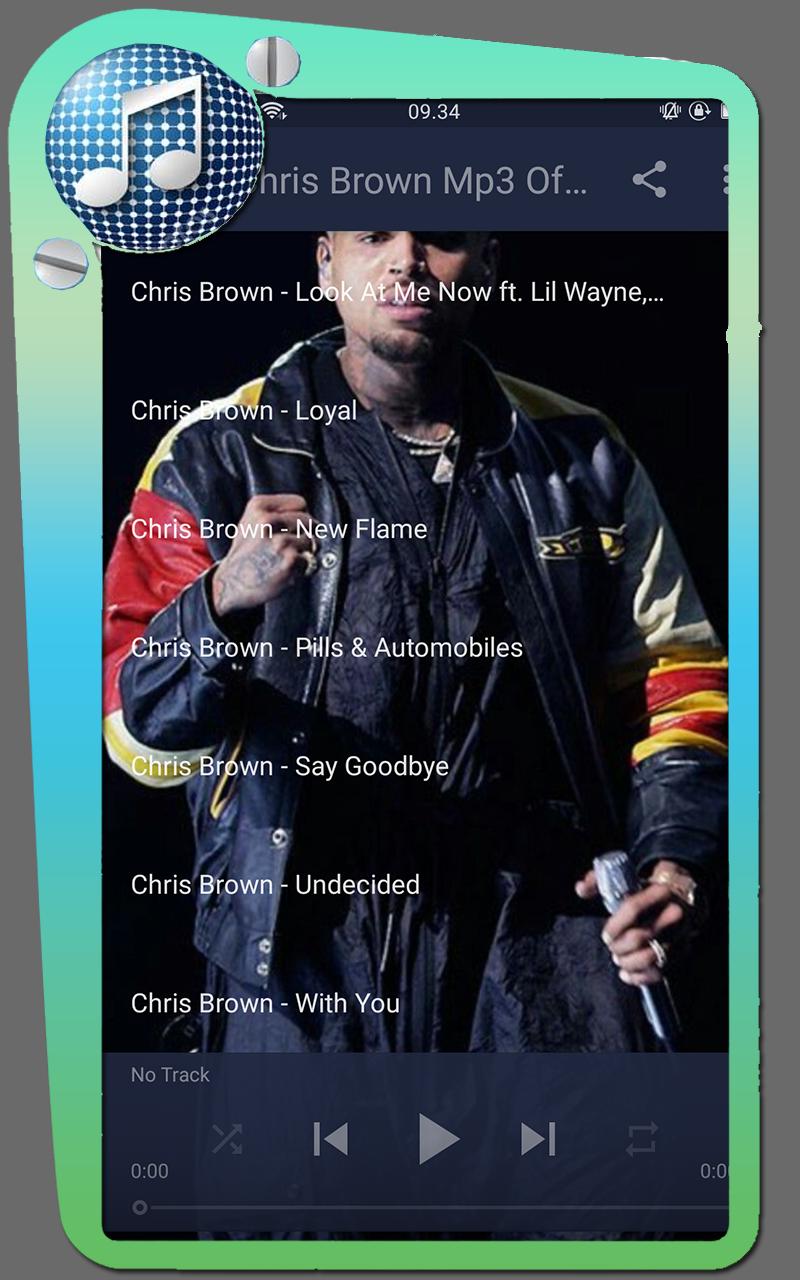The image depicts a smartphone screen against a gray background, resembling a screenshot. In the center of the screen is a photo of Chris Brown holding a microphone, dressed in a black jacket with multicolored sleeves. Above the image, the text "Chris Brown mp3" is displayed. 

In the upper left corner of the screen, there is a large circle with a music note icon inside, surrounded by several dots. Below Chris Brown's picture, at the bottom of the screen, a basic music player interface is visible, featuring a play button (triangle), and forward and backward buttons. The text "no track" appears in the upper left corner of this player section.

The phone's screen has a green border with two straight screws (resembling minus signs), one located below the music note circle on the left side, and the other above it on the right side. All of this is enclosed within a gray rectangular box.